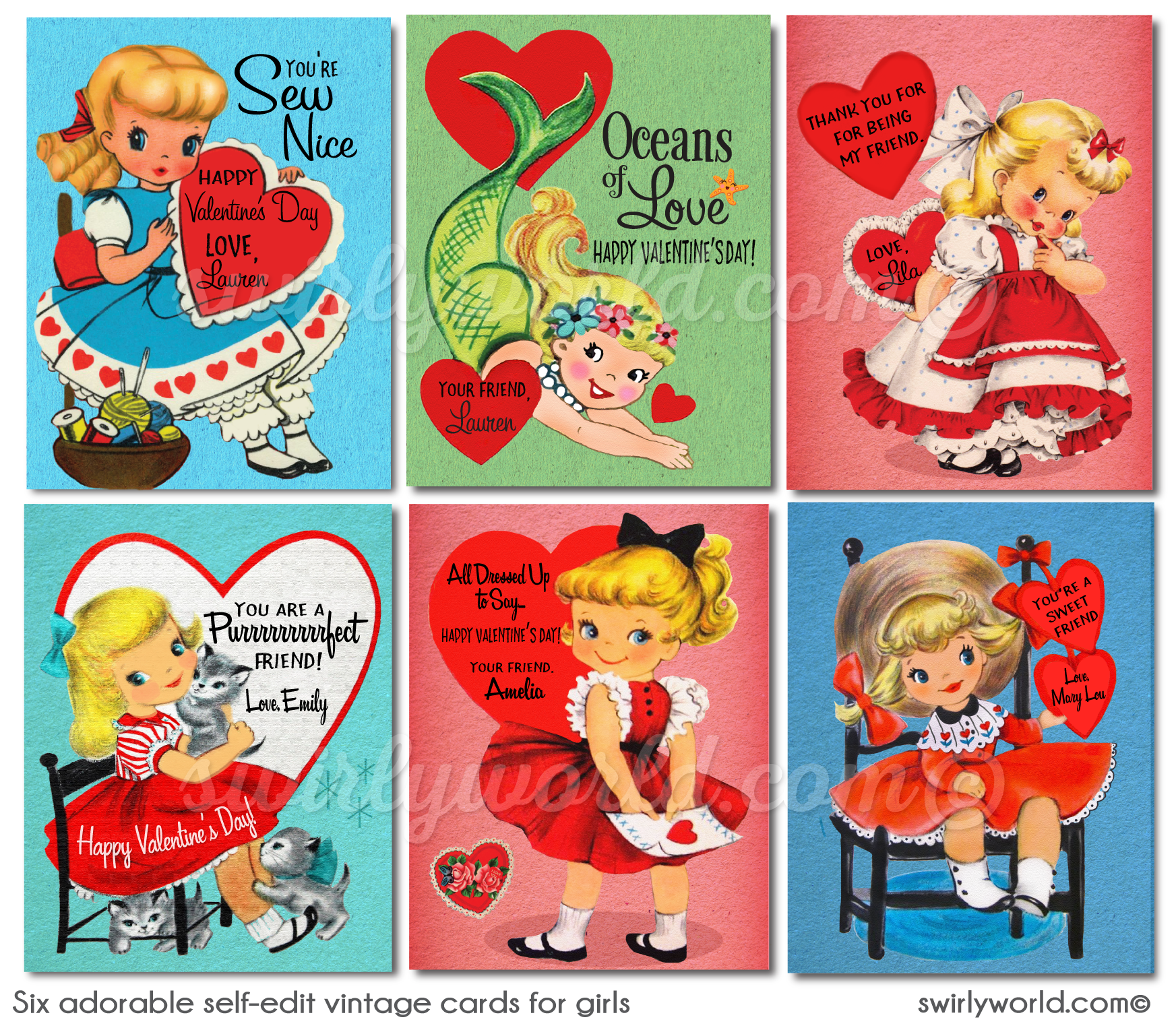This image showcases six vintage Valentine's Day cards from the 1950s, designed specifically for girls. Each charming card features a cartoon-like illustration of a blonde-haired girl with either ribbons or flowers adorning her curly locks. While five of the girls are depicted wearing pinafore-style dresses in shades of red, white, and blue, the girl in the top center card is depicted as a mermaid with a green fin. Each frame in the collage—arranged two rows high with three cards per row—is vibrant with backgrounds in blue, green, or red. The cards, slightly rectangular in shape and hand-colored with a watercolor-like quality, are adorned with red hearts and inscribed with personalized Valentine's messages such as "Oceans of Love, Happy Valentine's Day, your friend Lauren" and "You are a perfect friend, love Emily." The caption at the bottom left reads "six adorable self-edit vintage cards for girls," while "swirlyworld.com ©" appears in black on the bottom right. The primary color palette consists of blue, green, white, and yellow, capturing the nostalgic and playful essence of vintage school Valentine’s Day cards.